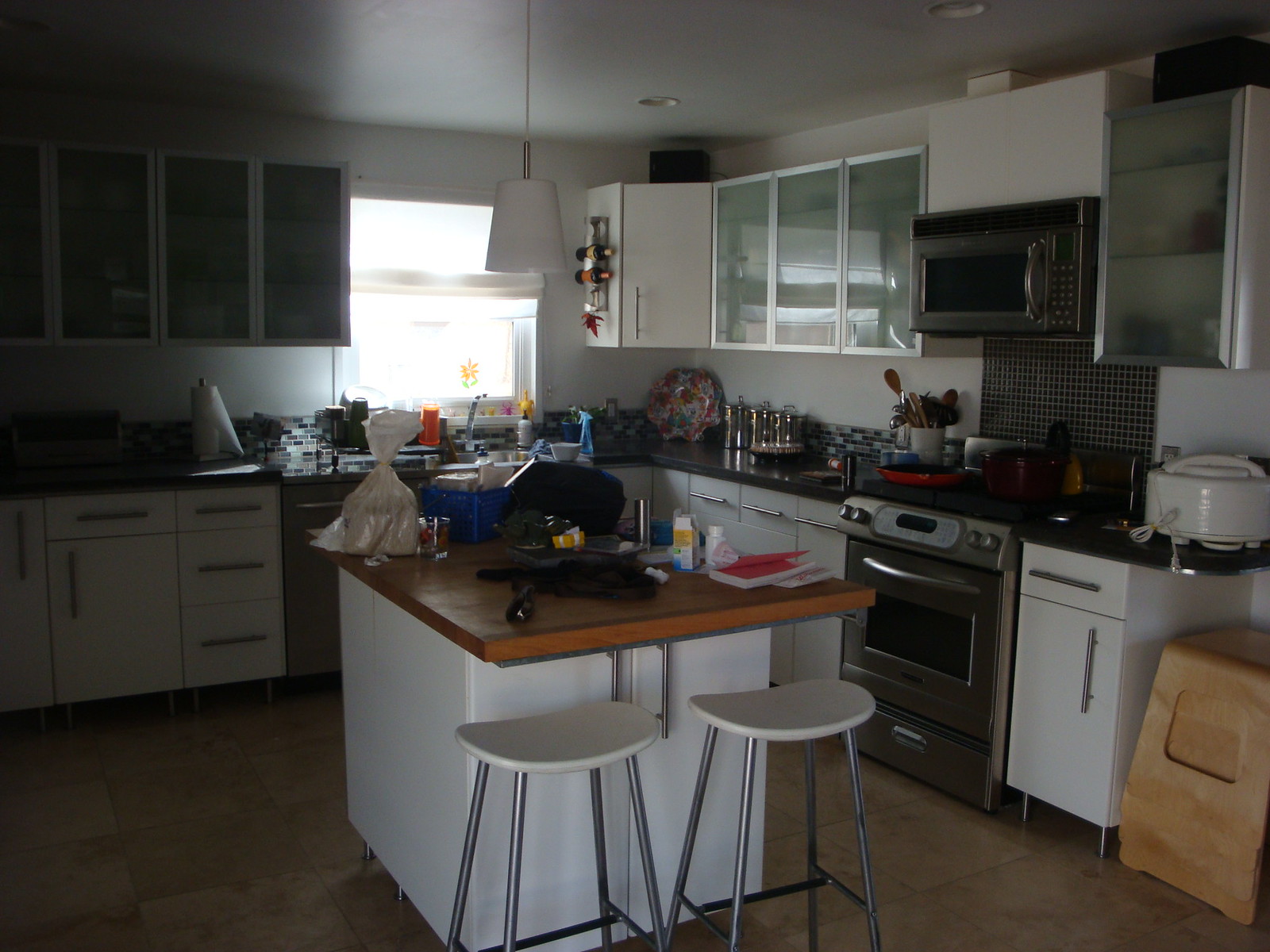In the dimly lit photograph of a kitchen interior, the space is illuminated solely by a large square window on the left wall, casting a diffused white light. The viewpoint captures the corner where the left and right walls meet, offering a glimpse of the kitchen's layout. The ceiling and all walls are uniformly white, creating a standard and clean appearance. Dominating the center of the room is a kitchen island with white sides and a contrasting wooden surface. In front of the island are two stools, each featuring a sleek white plastic seat supported by four chrome-finished metal legs. Along the left wall, four spacious cabinets provide ample storage, while the right wall is adorned with three cabinets, their translucent plastic or glass doors partially revealing the contents inside. A stainless steel stove with a distinctive black triangle detail occupies a prominent spot on the right wall, crowned by a built-in microwave that combines chrome and black finishes. The countertops near the stove are notably black, adding a touch of contrast to the predominantly white kitchen.